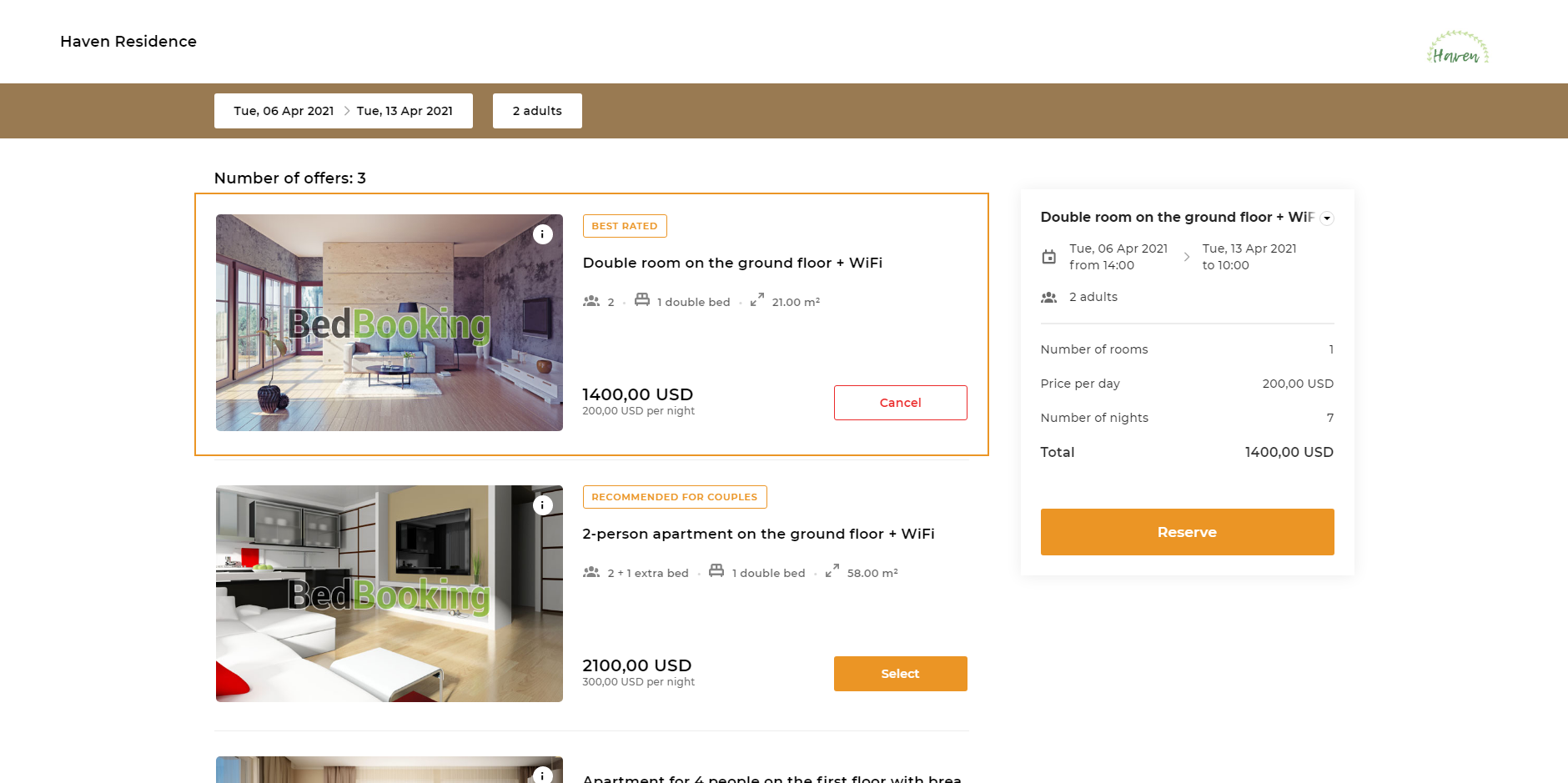This web page appears to be for rental properties or a bed and breakfast, although the exact name of the company is unclear. The company's name is indicated in green text on the right side of the page, while the left side features "Haven Residence" in black, which might be the property’s name. Beneath that, there is a brown bar where the user has entered their dates of interest and indicated that two adults will be staying. The search results show that there are three available options for the selected dates and two adults.

The top option is highlighted and gives a detailed view of a double room located on the ground floor. This option includes amenities such as Wi-Fi, accommodates two people, comes with a double bed, and provides information on the square footage and cost per night. Additional details, including the total cost, are displayed on the right side, and there is a prominent "Reserve Now" button in a large orange block.

The second option listed is a two-person apartment also located on the ground floor with Wi-Fi. This entry shows the number of beds, although some details are difficult to read, and lists the price at $2,100 per night. Similar to the first option, selecting this one would likely display more detailed information on the right side of the page.

A third offering is mentioned but requires scrolling down to view its details.